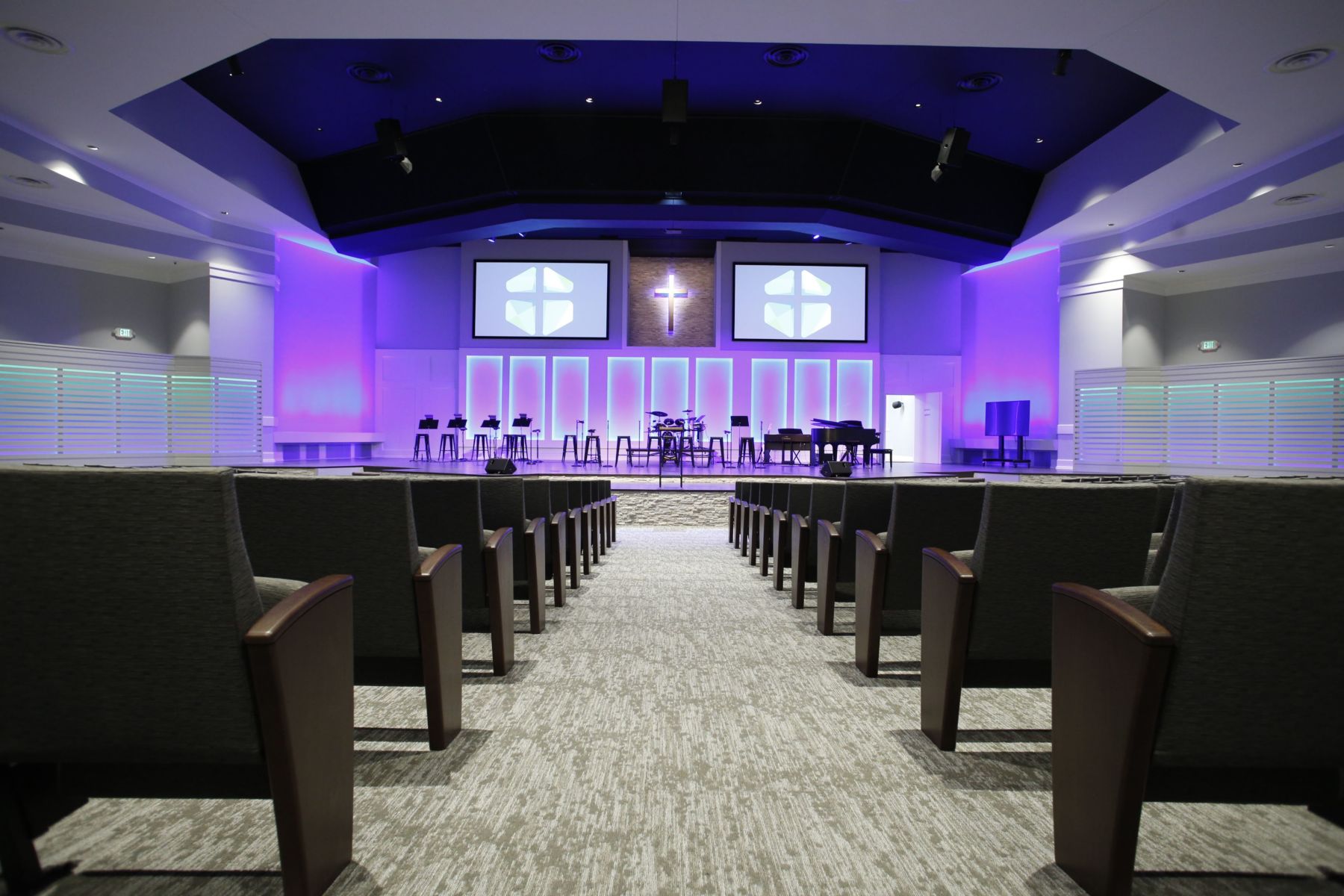This image captures the interior of a modern megachurch, where sleek design meets spiritual ambiance. The church features predominantly white walls and a recessed dark blue section in the center of the ceiling, which houses mounted lights directing soft illumination towards the stage. The perspective is down the center aisle, flanked by rows of pew chairs that resemble movie theater seats, upholstered in gray fabric with brown armrests. The carpet is a light gray with a speckled pattern of brown and gray.

The elevated stage, with white stonework on the sides and a shiny dark blue surface, is brightly lit with a soft lavender and muted neon hues of purple and blue. It hosts multiple chairs, a piano, and a podium, with places for a band and a choral line. Behind the stage on the back wall is a large illuminated cross, bathed in white and purple light, flanked by two prominent logos or screens. The overall modern and clean look is further accentuated by the absence of additional text or decorations, focusing all attention on the solemn yet inviting worship space.